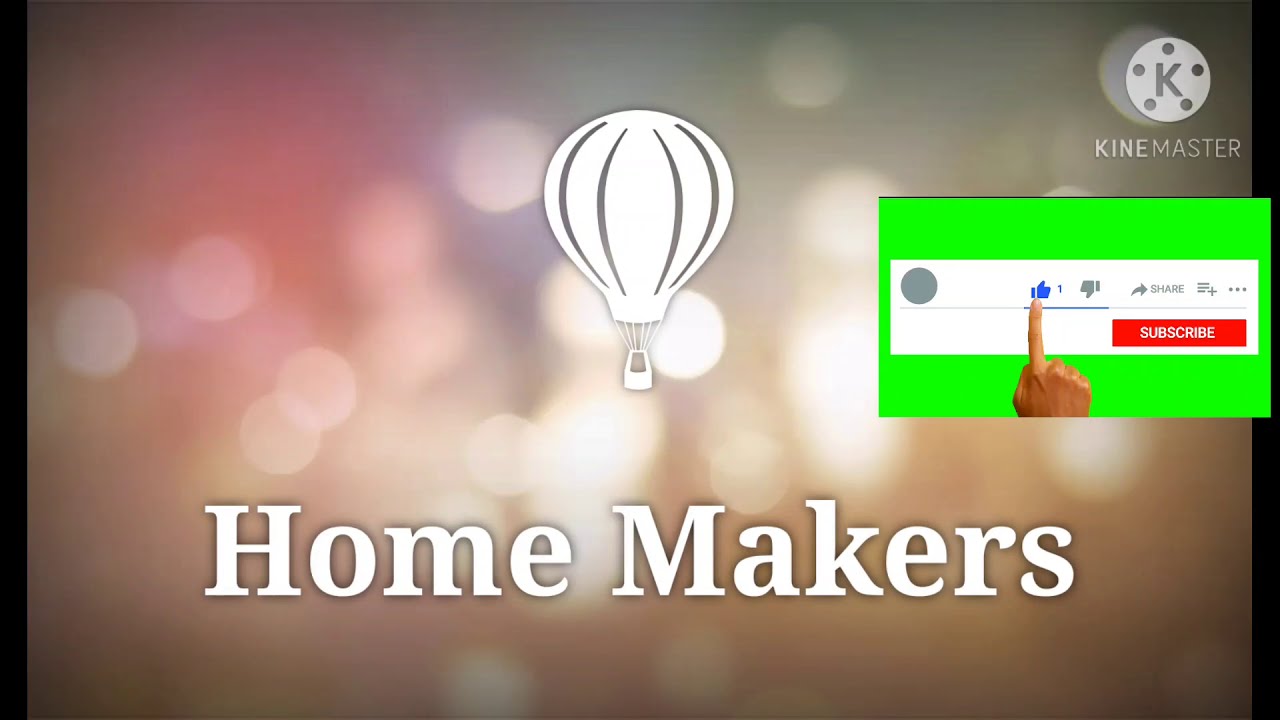In this image, a white hot air balloon is prominently centered, depicted as an outline with black lines adorning the middle and connecting downward to the basket. Directly beneath the balloon, the words "Homemakers" are boldly displayed in large, white letters. The background is a blur of white light circles, giving the impression of a softly illuminated scene.

The upper right-hand corner features a logo: a light gray circle with a "K" in the middle and small black dots encircling it. Below this logo is the text "KineMaster." Adjacent to this, on the right edge of the image, is a lime green rectangle containing a smaller white rectangle. This white rectangle houses several interactive icons, including a blue thumbs-up, a thumbs-down, a share icon, and a red "Subscribe" button. A hand with a pointing finger emerges from the bottom of the image, directing attention to the "Like" button. 

A black border frames the image on both the left and right sides, adding a stark contrast to the otherwise colorful and luminous background. The overall impression is of a vibrant yet orderly advertisement, with each element carefully placed to guide the viewer's attention.